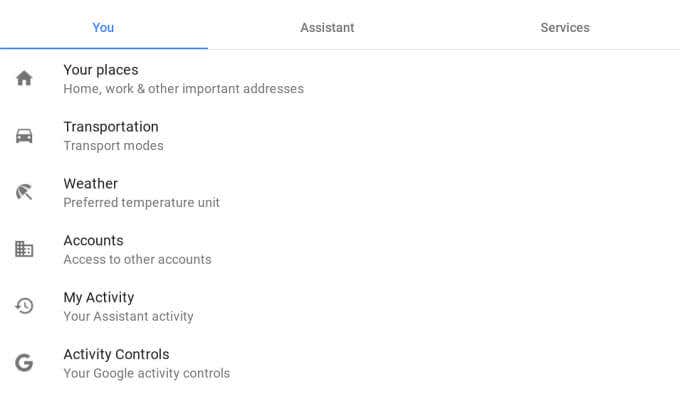Here is a detailed and cleaned-up version of the caption:

---

The image is a screenshot featuring a predominantly white background. At the top left corner, there is a blue vertical line with the word "YOU" written in blue font (Y-O-U) placed on top of it. Extending horizontally from the blue line is a gray line that spans the rest of the page. In the center of this gray line, the word "assistant" is written in gray font. To the far right, "services" is written, also in gray.

Below this horizontal section, the content is organized into a vertical column of sections, each featuring icons and descriptive text:

1. **Your Places**
   - Icon: A house.
   - Text: "Home, work, and other important addresses."

2. **Transportation**
   - Icon: A car.
   - Text: "Transportation modes."

3. **Weather**
   - Icon: An umbrella.
   - Text: "Preferred temperature unit."

4. **Accounts**
   - Icon: A graph.
   - Text: "Access to other accounts."

5. **My Activity**
   - Icon: A clock.
   - Text: "Your Assistant activity."

6. **Activity Controls**
   - Icon: A large 'G'.
   - Text: "Your Google activity controls."

All the text, apart from "YOU" at the top, is in black and gray font. The elements are neatly arranged in column format under the word "YOU." The background remains white throughout the entire page.